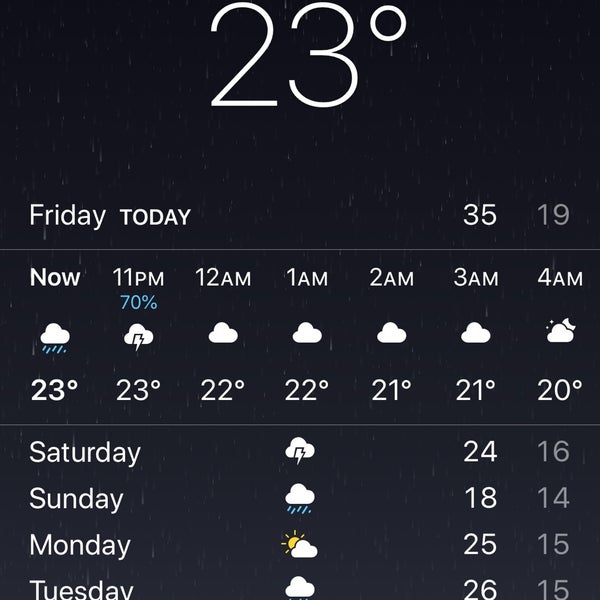The image depicts a detailed weather forecast for the upcoming week, with a clear and informative layout. In the top center, large bold text displays the temperature as "23°". The background features a night sky, dotted with white stars and lines, adding a celestial touch to the design.

On the mid-left, the word "Friday" is prominently displayed, followed by "today" and the numbers "3519". A thin horizontal white line spans the width of the image, separating the day's overview from hourly details.

The middle section shows specific time slots: "Now", "11pm", "12am", "1am", "2am", "3am", and "4am". Each time slot is accompanied by a cloud icon representing different weather conditions: the first cloud is raining, the second depicts thunder, the next four clouds are plain, and the last cloud features a sun partially obscured by it.

At the bottom, the days "Saturday", "Sunday", "Monday", and "Tuesday" are listed on the left, each with corresponding cloud icons indicating the forecast for those days. The image provides a comprehensive and visually engaging weather update.